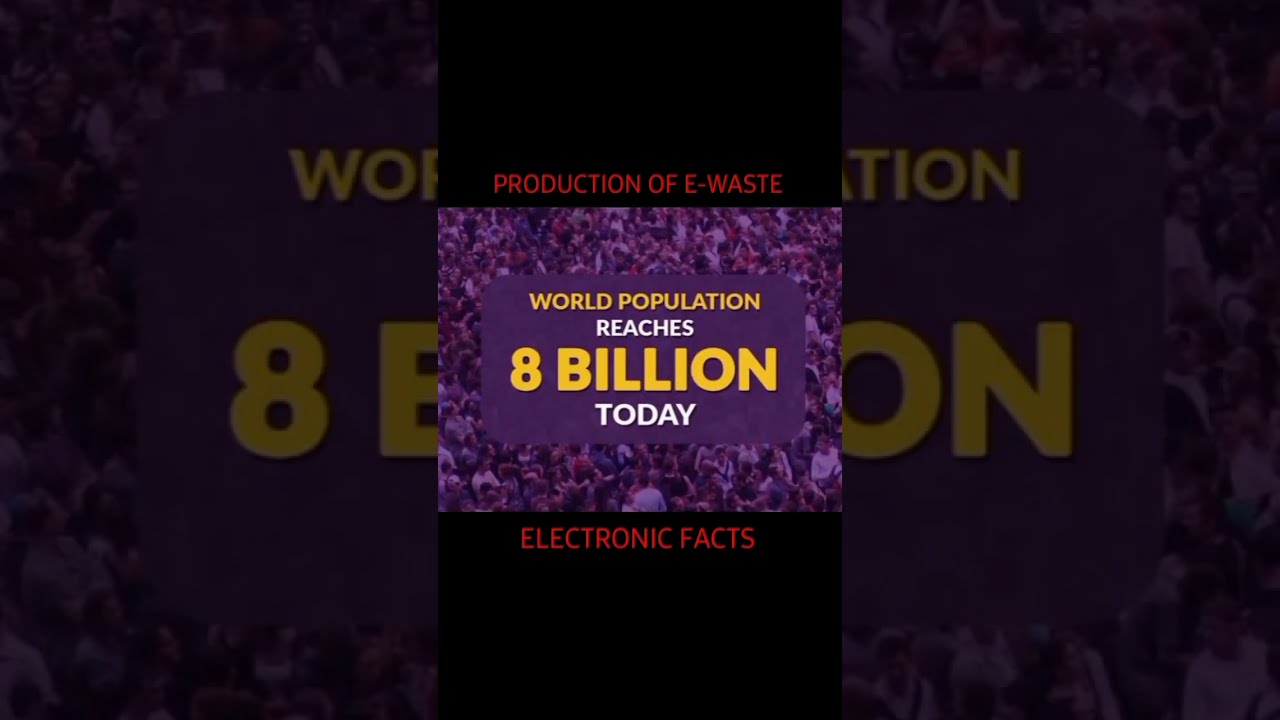This rectangular infographic, likely a screenshot from a social media app like TikTok or Instagram, captures a compelling visual message about global population. Measuring approximately six inches wide and three inches tall, the central focus is a crowded scene of people overlaid with hues of light purple. Dominating the center is a beveled, purple rectangle containing impactful text: "World Population" in gold print, "reaches" in white, "8 billion" in large gold letters, and "today" in white.

The image composition is structured into a top, center, and bottom section, with black backgrounds framing the top and bottom. At the top center, in red print, the text "Production of E-Waste" is displayed, and at the bottom, also in red, "Electronic Facts." The primary central image is flanked by larger, darker copies of the crowd scene, creating a cohesive and visually engaging effect. The graphic's color palette includes black, red, purple, pink, yellow, white, and gray, enhancing its striking and informative presentation. In essence, the design underscores the announcement of the world population reaching 8 billion, juxtaposed with a pertinent commentary on e-waste production.